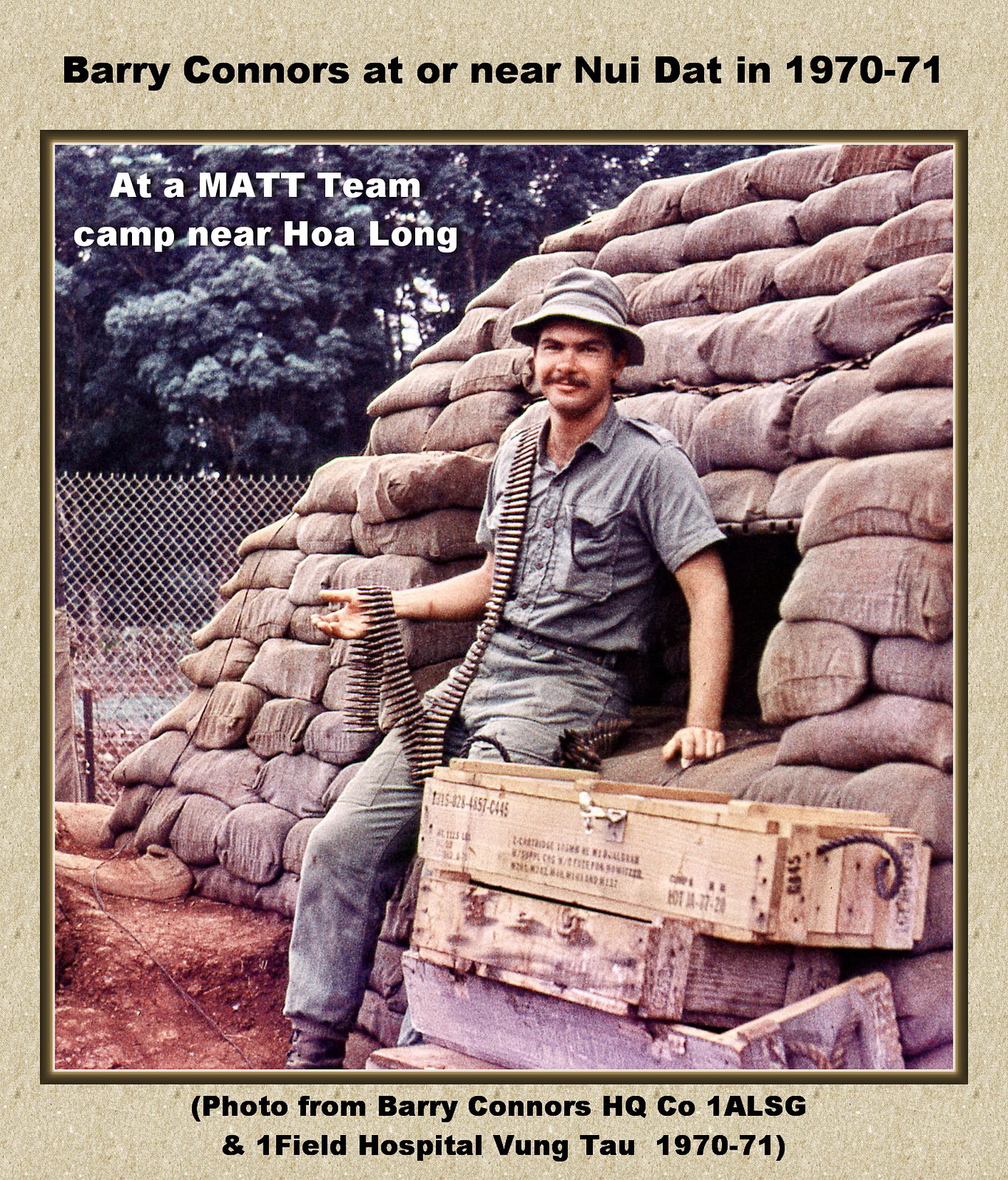The image captures a man, likely a soldier during the Vietnam War, leaning on a constructed wall of brown sacks, resembling a makeshift bunker. His attire is uniformly gray, consisting of a short-sleeved button-down shirt, long pants, and a hat, entirely military in appearance. He wears brown combat boots and a belt of machine gun bullets draped over his right shoulder, with the end wrapped around his right hand, while his left hand and body rest on top of the sacks. The ground beneath him is dirt, and a chain-link fence along with some trees are visible in the background. Wooden crates are positioned in the lower right-hand corner of the image. Text on the photo provides the context: "Barry Connors at or near Nui Dat in 1970-71" at the top, "at a MAT team camp near Hoa Long" in the upper left corner of the photo, and "photo from Barry Connors HQ CO1ALSG and Onefield Hospital Vung Tau 1970-1971" at the very bottom in black text. The man appears to be slightly gritting his teeth and is looking toward the camera, positioned at an angle akin to the 7 o'clock direction.